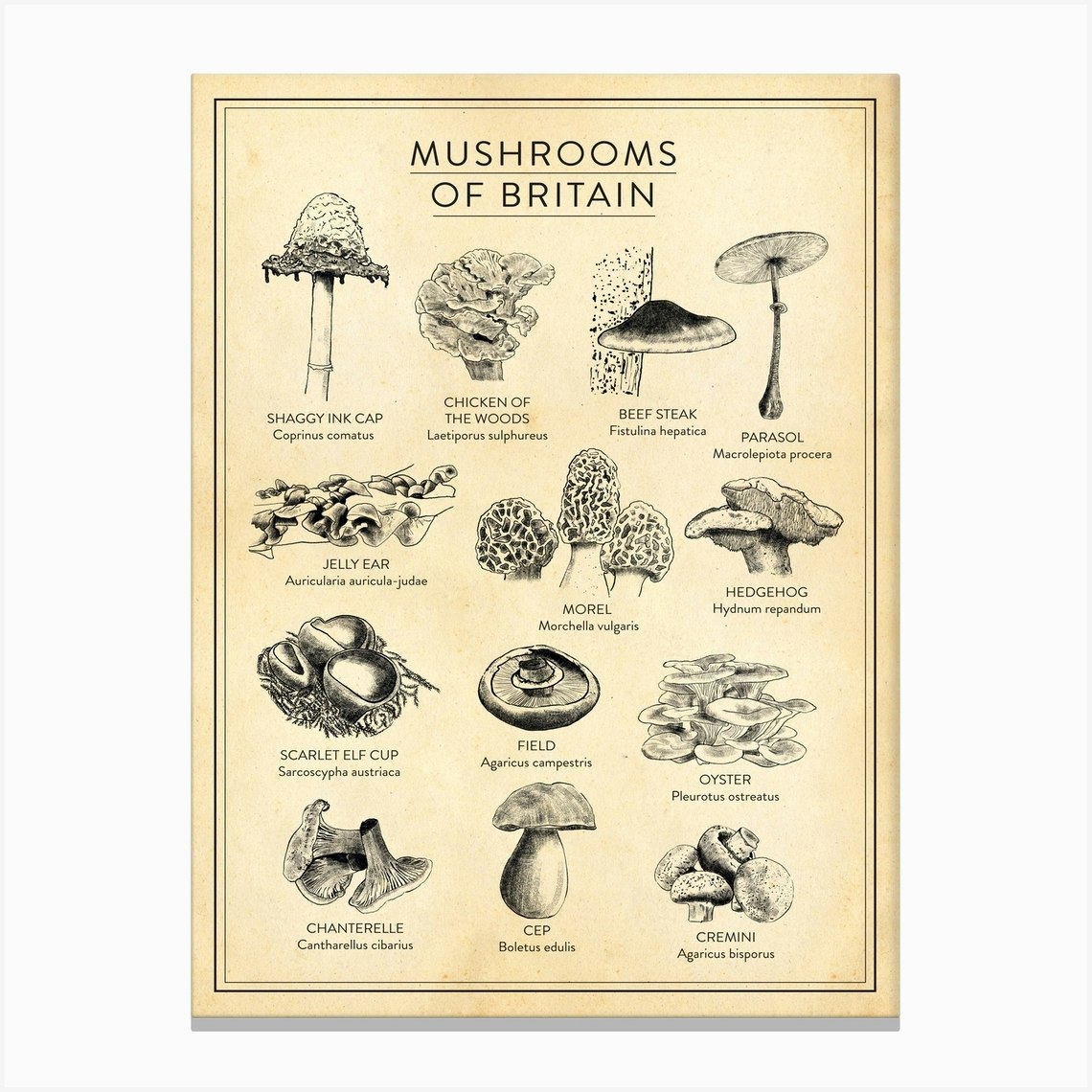The image showcases a vintage, weathered poster titled "Mushrooms of Britain," presented in a portrait orientation. The title is prominently displayed at the top in black, underlined text with a double underline for emphasis. The poster features detailed black-and-white line art drawings of various mushroom species, each labeled with their common and scientific names. The illustrations are arranged in four rows against a beige background that adds a sepia-toned aesthetic, emphasizing the vintage feel.

Starting from the upper left corner, the first row includes:
1. Shaggy Ink Cap (Coprinus comatus) - depicted with its characteristic shaggy hat-like cap.
2. Chicken of the Woods (Laetiporus sulphureus) - illustrated with rosette-shaped clusters.
3. Beefsteak (Fistulina hepatica) - shown growing shell-like on the side of a tree.
4. Parasol (Macrolepiota procera) - notable for its umbrella-like shape.

The second row features:
1. Jelly Ear (Auricularia auricula-judae) - with its ear-like appearance.
2. Morel (Morchella vulgaris) - depicted with a honeycomb-like cap.
3. Hedgehog (Hydnum repandum) - identifiable by its spiky undercap.

The third row displays:
1. Scarlet Elf Cup (Sarcoscypha coccinea) - with its bright, cup-shaped fruiting body.
2. Field Mushroom (Agaricus campestris) - classic and well-known among mushroom foragers.
3. Oyster Mushroom (Pleurotus ostreatus) - with its fan-shaped cap.

The final row includes:
1. Chanterelle (Cantharellus cibarius) - renowned for its trumpet-like structure.
2. Cep (Boletus edulis) - also known as King Bolete, illustrated with its stout stem and large cap.
3. Cremini (Agaricus bisporus) - the familiar button mushroom in its mature form.

The entire illustration is bordered with a black double-line frame, and the poster itself is set against a light gray background, highlighting its classic and educational design.